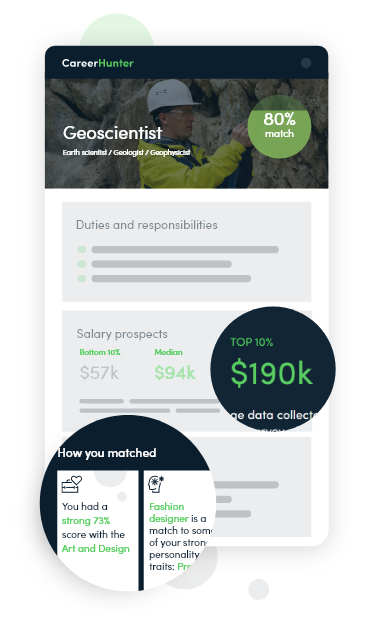### Captivating Career Advertisement for Geoscientist with Comprehensive Details

The image appears to be a high-quality screen capture, likely intended for an advertisement promoting career opportunities. At the top, the banner displays the text "Career Hunter" in bold green and white font. Below this, the partial view of a green circle is visible against a navy background.

Taking center stage in the image is a professional-looking man clad in a yellow jacket, wearing a white hard hat and protective goggles. The caption "Geoscientist" is written in white font prominently next to him.

Further down, the text includes several sections with various details:

1. **Match Information:**
   - A green circle with the text "80% match" indicating the suitability for the position.
   
2. **Details of Duties and Responsibilities:**
   - A gray box encapsulates this section, listing specific job functions accompanied by green bullet points.

3. **Salary Prospects:**
   - A detailed breakdown highlighted in green and navy:
     - Bottom 10%: $57K
     - Median: $94K
     - Top 10%: $190K

Continuing down, another navy and white circle appears, labeled "How You Matched." Two white boxes provide further insights:

1. **Art and Design Compatibility:**
   - The first box has a shopping bag icon with a heart and states, "You had a strong 73% score with the art and design," in black and green font.

2. **Personality Traits and Job Match:**
   - The second box, featuring a small head-of-a-person icon, notes that "Fashion Designer is a match to some of your strong personality traits."

The image ends with partial white text that is cut off, leaving the remaining details indiscernible. The overall visual quality of the image is clear, providing a comprehensive and engaging overview of the career information presented.